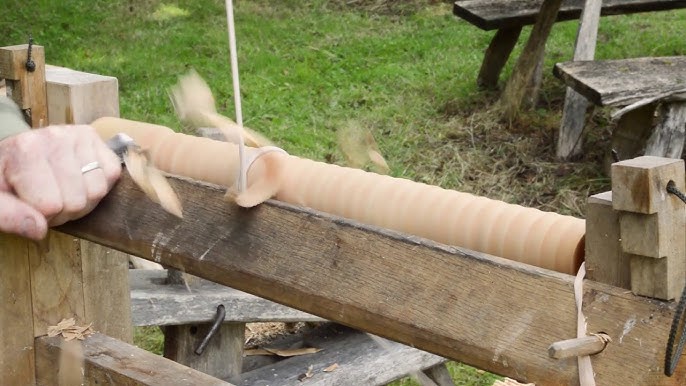A skilled carpenter is shown operating a lathe, meticulously shaping a cylindrical wooden pole. The pole, securely fastened between two clamps on either side of the machine, spins rapidly, creating a continuous blur of motion. The carpenter, wielding a sharp carving tool, expertly applies it to the revolving wood, effortlessly carving intricate designs with precision. The spinning action of the lathe facilitates the cutting process, allowing the wood to be evenly and smoothly sculpted, achieving results that would be time-consuming and less refined through manual techniques alone. The scene captures the fusion of traditional craftsmanship with the efficiency of mechanized tools.